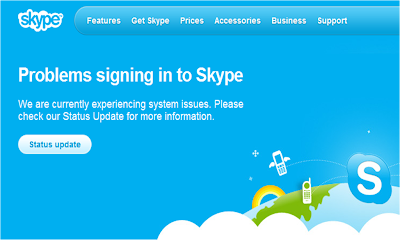The webpage for Skype features a light blue background with a white cloud in the top-left corner where the word "Skype" is prominently displayed in blue letters. A blue navigation bar below this includes the options: features, get Skype, prices, accessories, business support, and more. At the center of the page is a prominent message informing users of a current issue: "Problem signing into Skype. We are currently experiencing system issues. Please check our status update for more information." To provide further details, a white button with blue text allows users to check the status update.

In the bottom right-hand corner, there are several whimsical elements, including clouds, an image of Earth as viewed from space, giving it a spherical, "globy" appearance. The Skype logo is floating nearby, alongside a phone with wings, and another phone floating independently. A rainbow arches across the sky in the background, accompanied by several stars, offering a surreal and colorful visual experience. Overall, this page serves as a notification that the Skype service is currently down and provides a direct link for users to check the latest status updates.